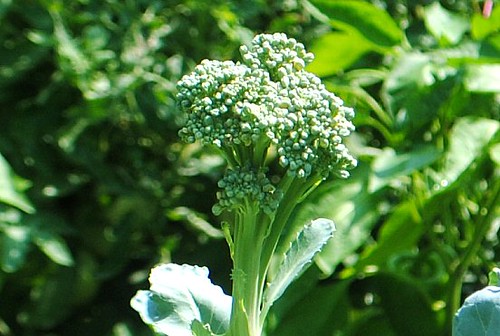In this brightly lit daytime photograph, the focus is on a vibrant broccoli plant standing prominently against a softly blurred background of mixed green foliage. The intense sunlight illuminates the scene, casting dense shadows and making the broccoli's leaves appear a light, almost pale green, contrasting with the darker green hues of the surrounding vegetation. The main broccoli stalk rises robustly, transitioning from a thick stem to several smaller clusters that resemble little bouquets of tiny green balls at the ends, almost like miniature trees. Despite the blur, the background reveals a hint of more green crops, emphasizing the solitary, healthy, and flourishing broccoli plant in the foreground.